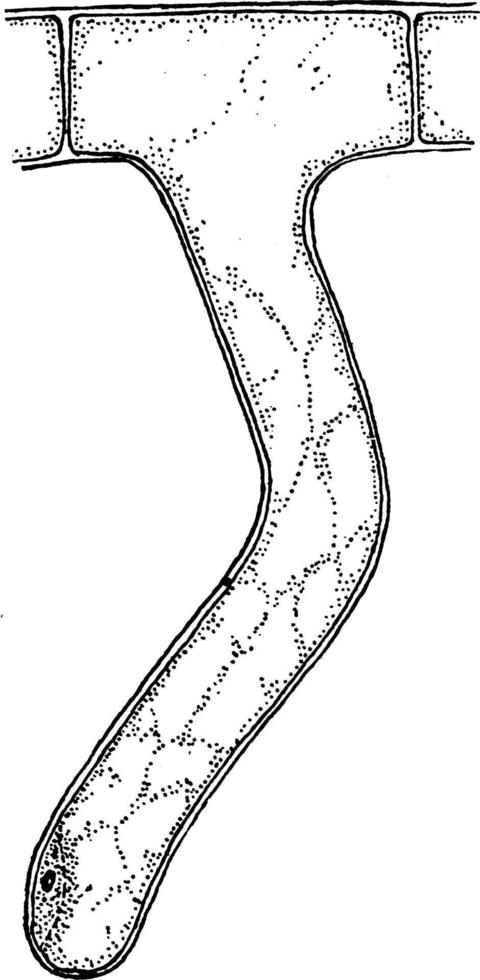This black-and-white illustration depicts a complex, snake-like structure that resembles a crooked, T-shaped pathway or tunnel system. At the top, the path branches horizontally on either side into two distinct blocks that converge into a larger, singular block, separated by what appears to be a thin wall or membrane. This top section is designed with stone-like paver textures.

From this larger block, the path extends downward, curving first to the right and then back toward the left, resembling a winding appendage akin to a snake, complete with a dark, eye-like spot near its tip. The entire structure is outlined with bold black lines, some featuring spaced intervals, creating a layered, detailed border. Throughout the illustration, numerous black dots scatter across the interior and around the eye-like spot, forming a web-like pattern. Enhanced by the intricate use of pen ink, the drawing suggests an organic or biological form, possibly indicative of a skin, organism, or vein-like system.